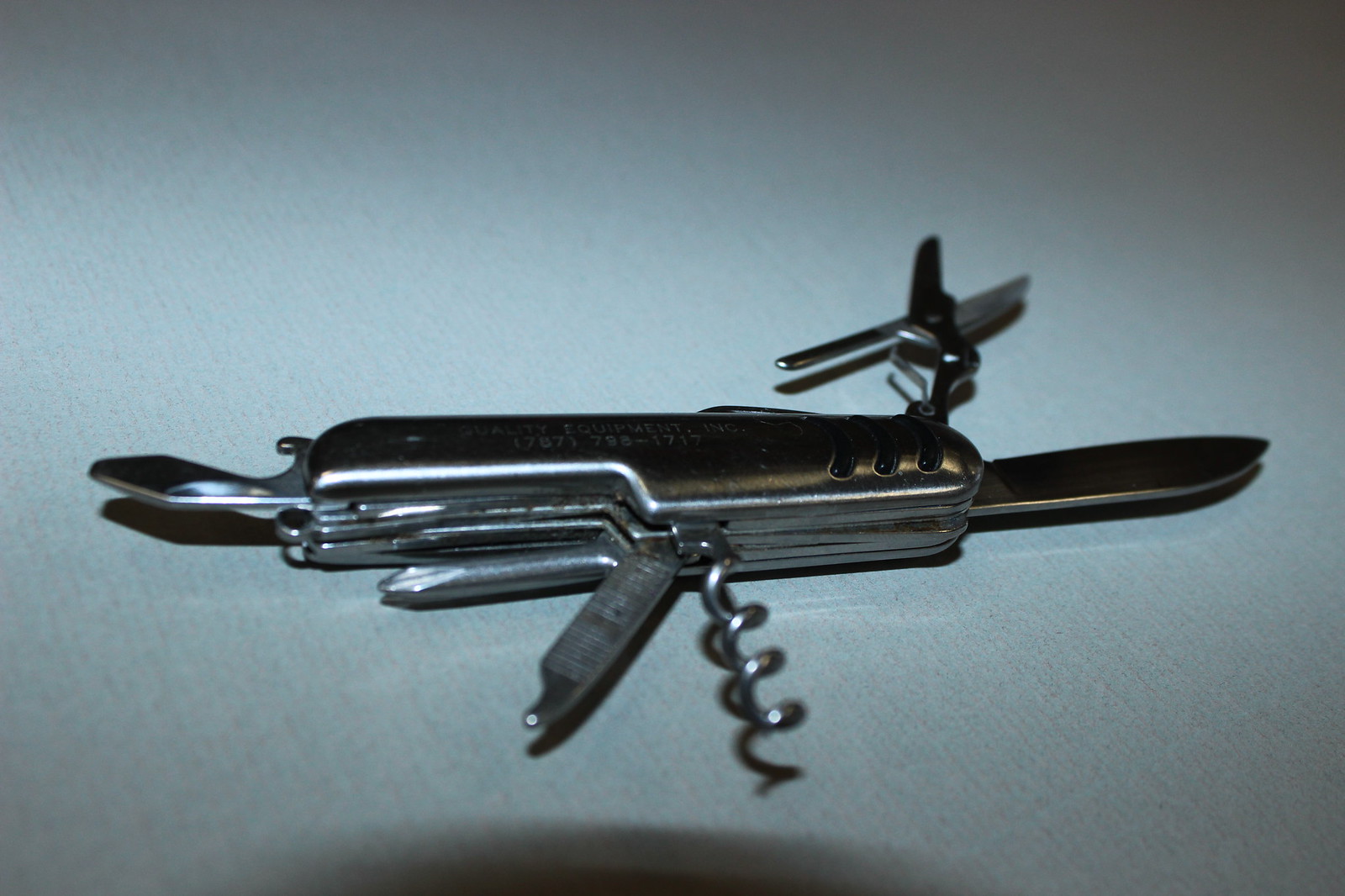This detailed photograph captures a Swiss Army-style pocket knife with a light silver metallic finish, set against a light blue, grainy background, possibly a painted table or textured paper. The image seems to have been taken with a camera flash, as reflections on the knife are visible, adding a dynamic light effect. The knife is intricately designed, featuring multiple extended tools. From left to right, there's a short knife blade, a corkscrew, a nail file, and a Phillips head screwdriver. Further down, there's a pair of fingernail clippers, another screwdriver head, a pair of scissors, and a bottle opener designed for pop or beer bottles. The knife measures approximately six inches in width and has distinctive writing at the top, indicating some equipment specifications and numbers, adding to its utilitarian character.